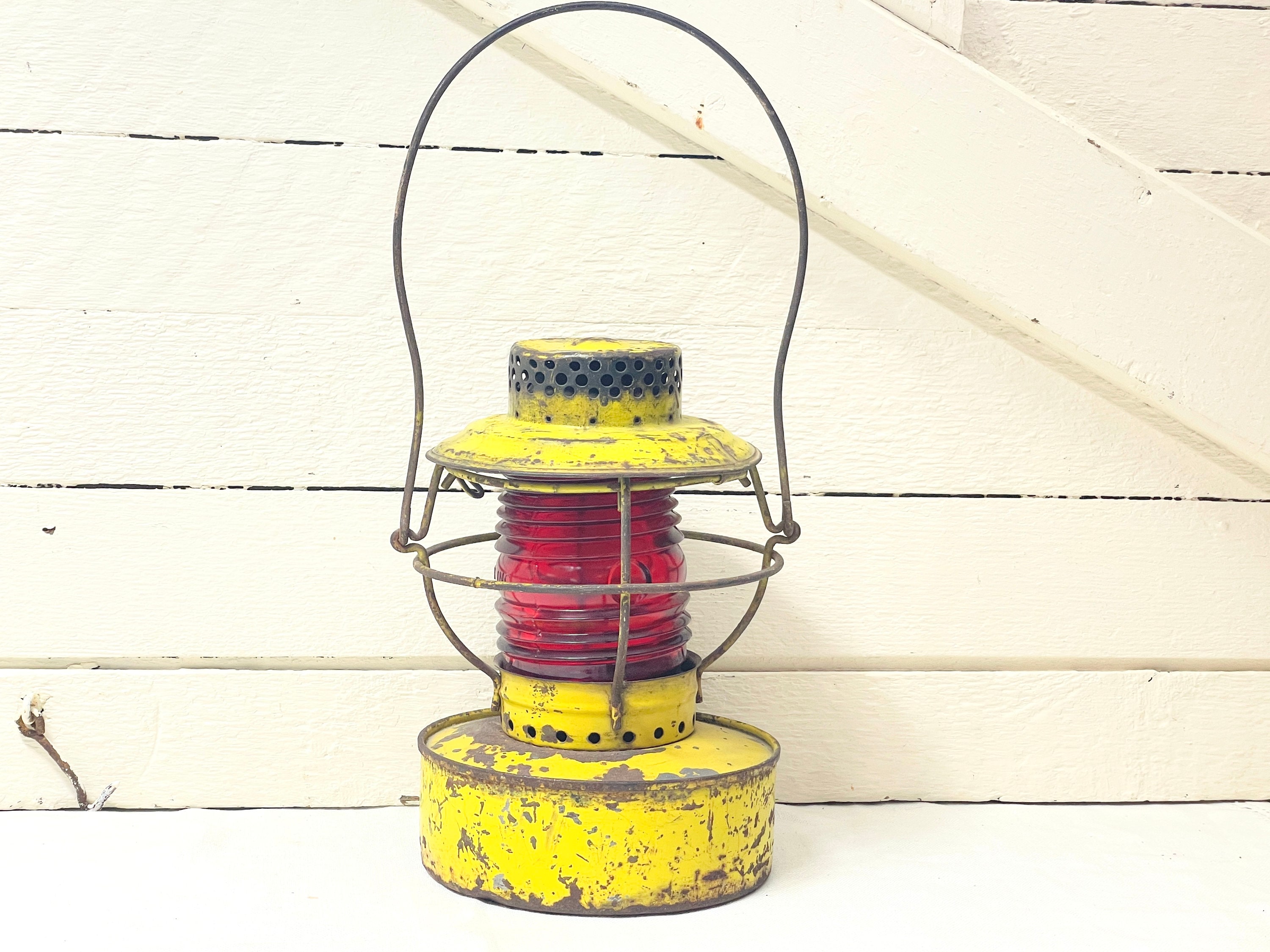The photograph features an antique lantern prominently positioned against a white-painted wooden background, which resembles either barn walls or a fence with narrow, black-lined slats. The lantern, painted in a bright but weathered yellow, shows considerable signs of age with extensive rust and patches of brown where the paint has chipped away. The central glass globe of the lantern is a striking red, encased by a metal cage. The lantern’s handle, constructed from the same metal as the cage, arches over the top, adding to its aged, rustic appearance.